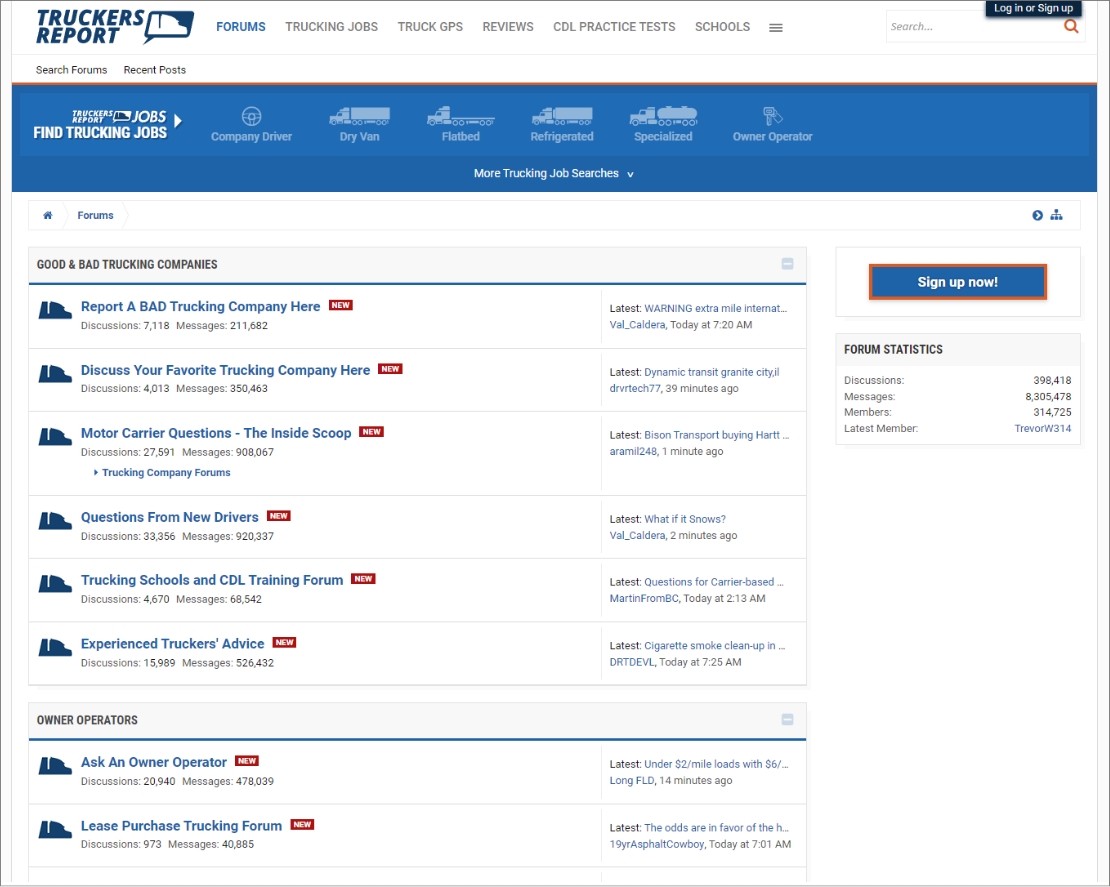The image showcases a webpage from the website "Chukar's Report." The header, set on a white background, prominently features the website's name and logo in dark blue font located at the top left corner. Adjacent to the site name, six categories are displayed: Trucking Jobs, Truck GPS, Reviews, CDL Practice Tests, Schools, and Forums, with the Forums category highlighted in blue, while the others are in grey. Next to the Schools category, stacked horizontal lines likely denote a menu option, followed by a search box. Above the search box, a dark blue banner with white font offers options to "Log In" or "Sign Up."

Beneath the header, options to "Search Forums" or "Recent Posts" are available. A broad blue section spans across the page, labeled "Jobs," with the subtitle "Find Trucking Jobs." This section includes tabs for various job types: Company Driver, Dry Van, Flatbed, Refrigerated, Specialized, and Owner-Operator, along with additional truck driving job searches.

The main content area shows the user navigating the Forums section, which includes categories like "Good and Bad Trucking Companies," with multiple related posts, and "Owner-Operators," featuring various discussions. On the right side of the page, a blue button outlined in orange, with white text, invites users to "Sign Up Now." Below this, a white box presents Forum Statistics, providing details on discussions, messages, members, and the latest member.